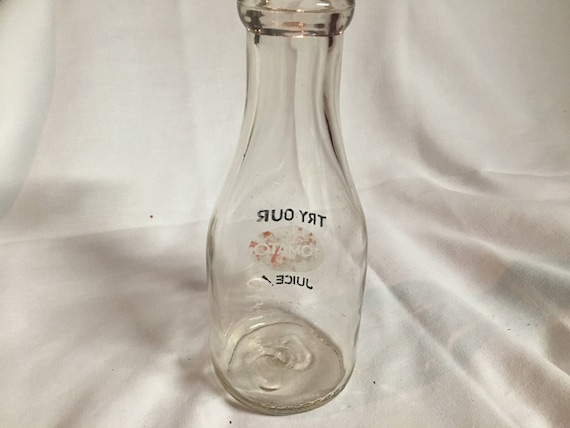This is a close-up photograph of a vintage glass bottle, potentially from the 1920s or 1930s. The bottle is relatively tall and features a clear, see-through design. The glass is thick, especially around the rim. Etched into the glass are several pieces of text that appear reversed in the photo. The most prominent words are "try our juice" and "tomato," suggesting a label or branding related to juice. The text is in white, framed by two sets of black text. The entire photograph is set against a backdrop of a white sheet or curtain, which is visibly wrinkled and extends from the base of the bottle to the top of the image. The well-lit room casts reflections and shadowing on the sheet, with some subtle coloring, including brown and a bluish-green shadow on the right side. The sheet also reflects parts of the bottle, enhancing the vintage aesthetic of the scene.